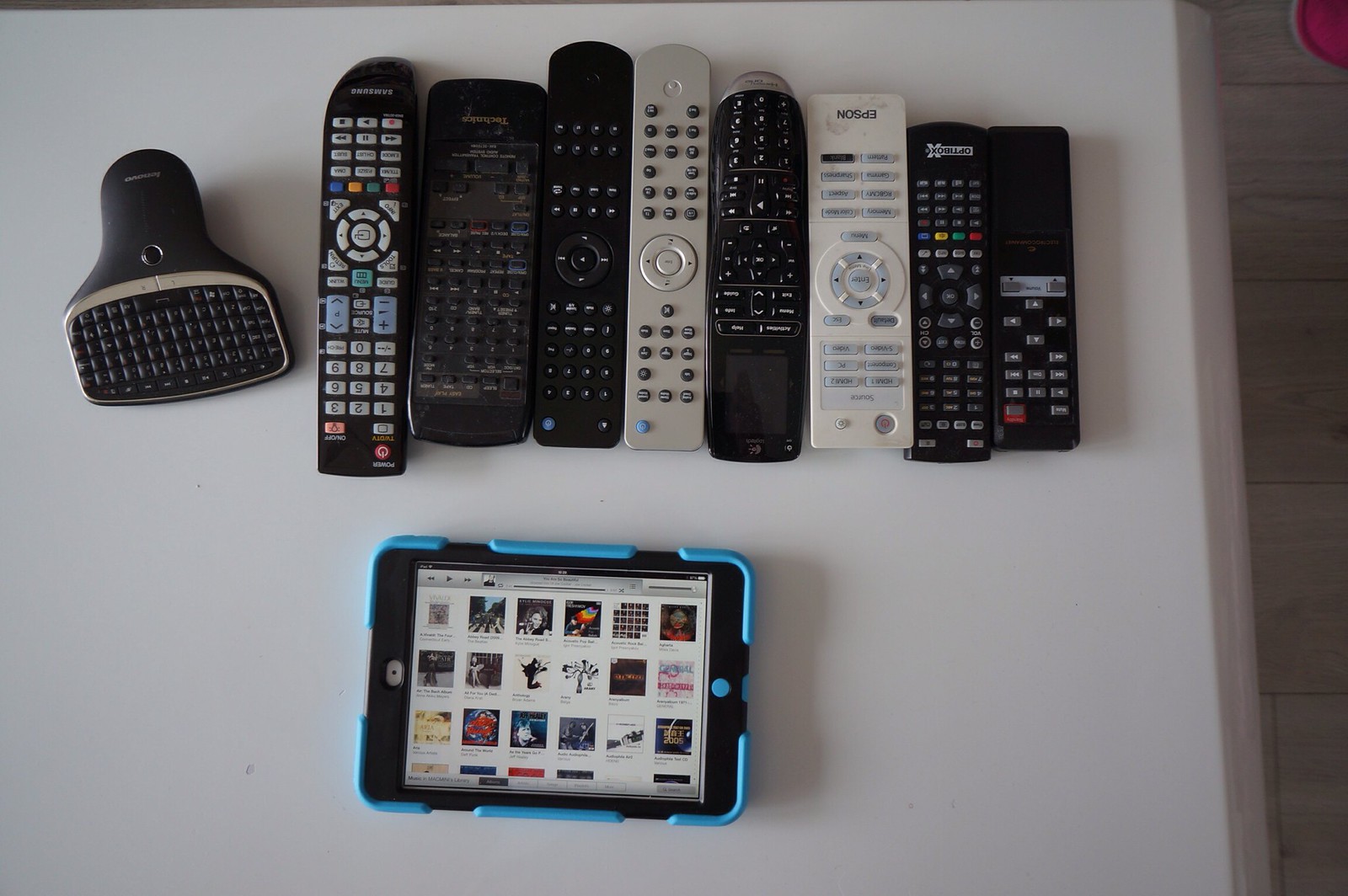This photograph captures an indoor setting featuring a collection of electronic devices meticulously arranged on a white folding table. Dominating the image are nine remote controls of varying shapes, colors, and conditions. These remotes, in hues of black, white, and silver, display a range of wear and tear, with some looking older and dustier than others. Positioned in a line above a distinct small tablet, the remotes share rectangular shapes and typically have white buttons. Notably, the tablet at the bottom of the image is encased in a bright blue and black protective rubber case and displays a music store interface with record albums. Adding to this assortment, a peculiar black device resembling an old BlackBerry with a small keyboard sits to the left, suggesting a bygone era of technology. All these items are set against the clean, white backdrop of the table, offering a detailed glimpse into a collection of electronic relics and contemporary gadgets.